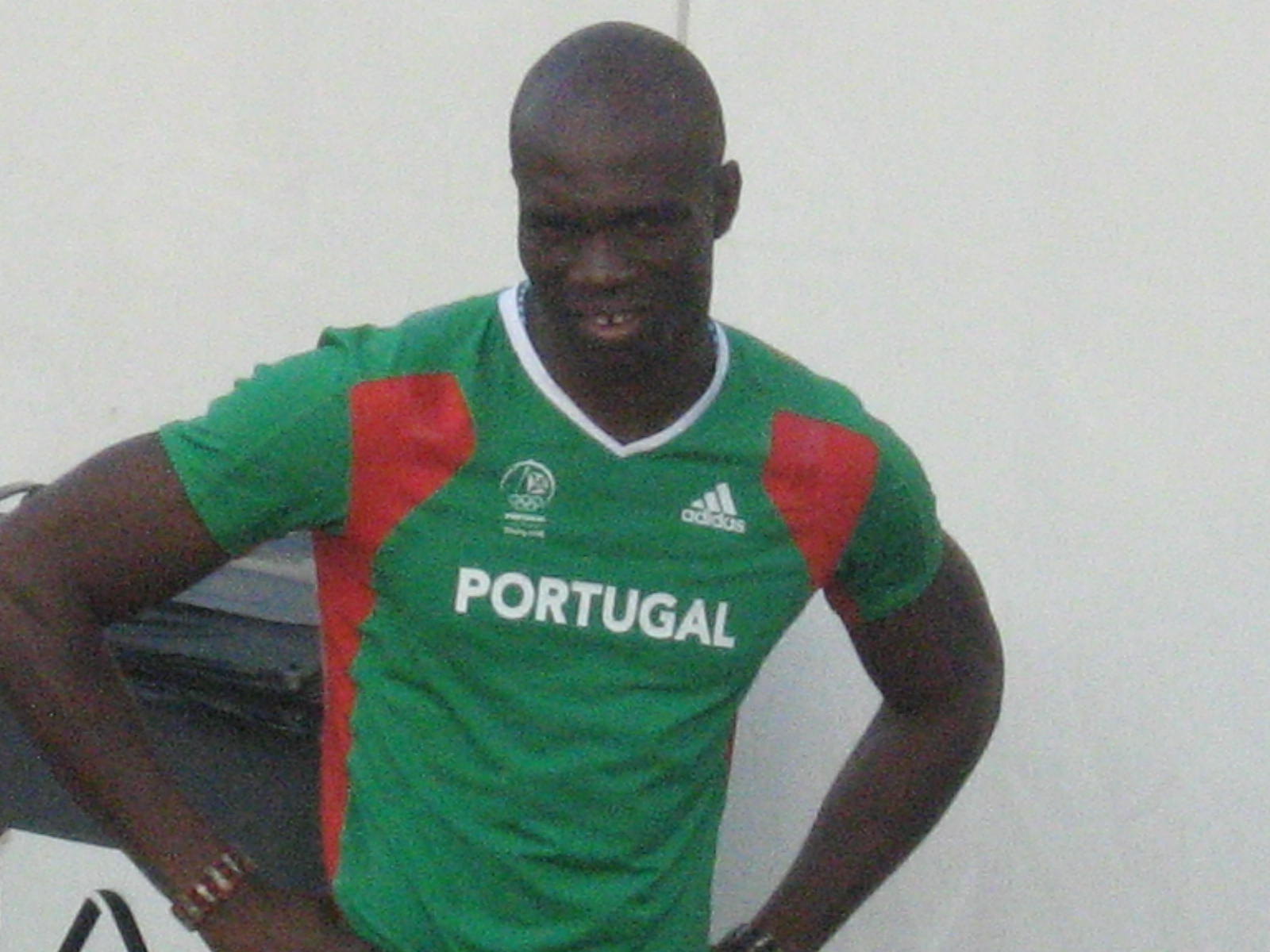The image depicts a darker-skinned, clean-shaven man with a bald head, dressed in a green jersey accented with red from the shoulders, under the armpits, and down the sides. The front of the jersey features the word "Portugal" in white, along with the Adidas logo on the left breast and another symbol, possibly related to the Olympics, on the right breast. The shirt has a v-neck with white trim. The man is standing with his hands on his hips, displaying a bracelet on each wrist. His posture reveals a slight grin, showing a noticeable gap between his front teeth. He is positioned against a white wall, with his head inclined slightly, causing his right ear to be out of view. The image is slightly blurry, compromising the clarity of finer details.